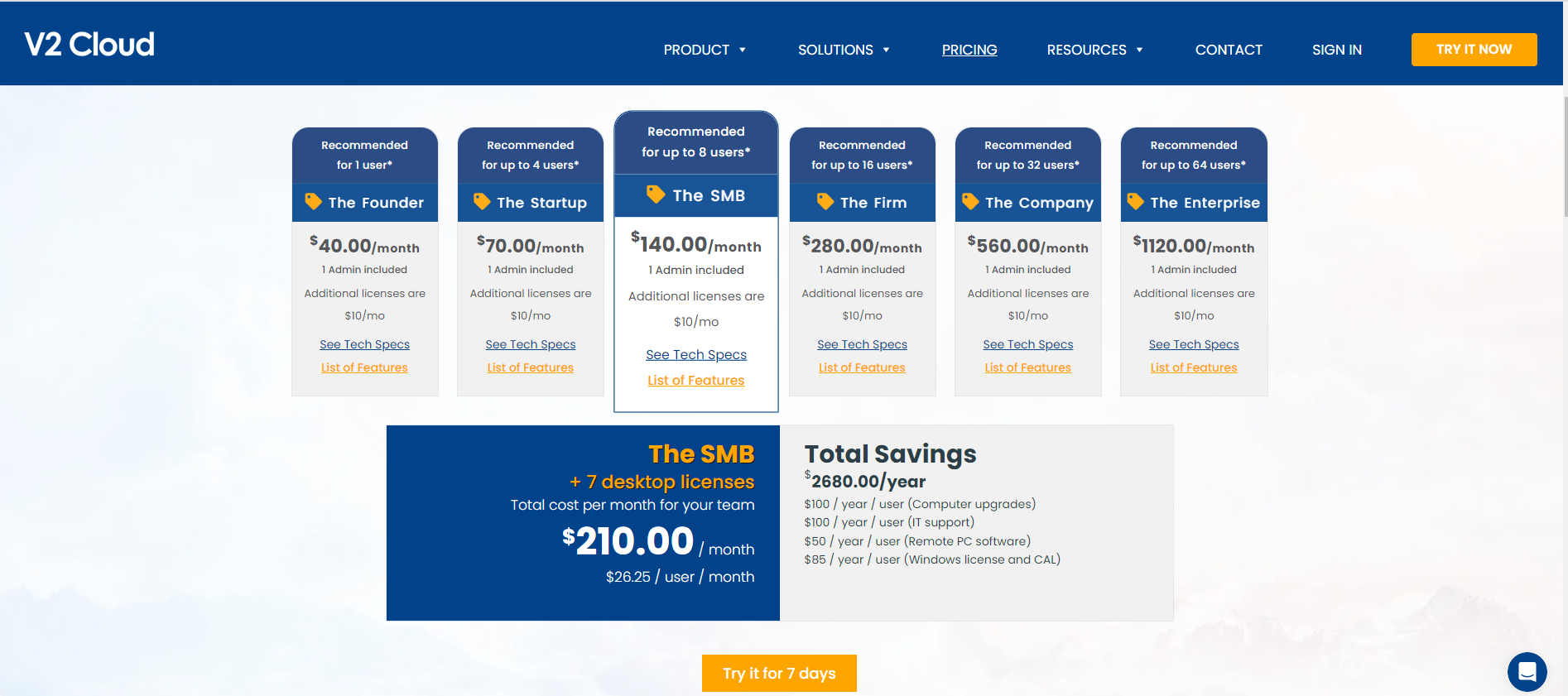The web page features a sophisticated layout on a light gray background, highlighted by a prominent blue banner at the top with crisp white lettering. Displayed in bold, "V2 Cloud" announces the name of the company on the left side of the banner. Adjacent to this, a series of navigational options such as "Product Solutions," "Pricing," "Resources," "Contact," and "Sign In" are clearly listed as drop-down menus, offering seamless navigation through the site. On the far right, a striking yellow button with white lettering invites users to "Try it now."

Beneath this cohesive banner, the page presents an array of examples illustrating the various services and products available for purchase from the company, complete with detailed pricing information. Concluding the page's content, a second yellow button marked with "Try it for seven days" in white lettering provides a clear call-to-action, encouraging potential customers to engage with the company's offerings.